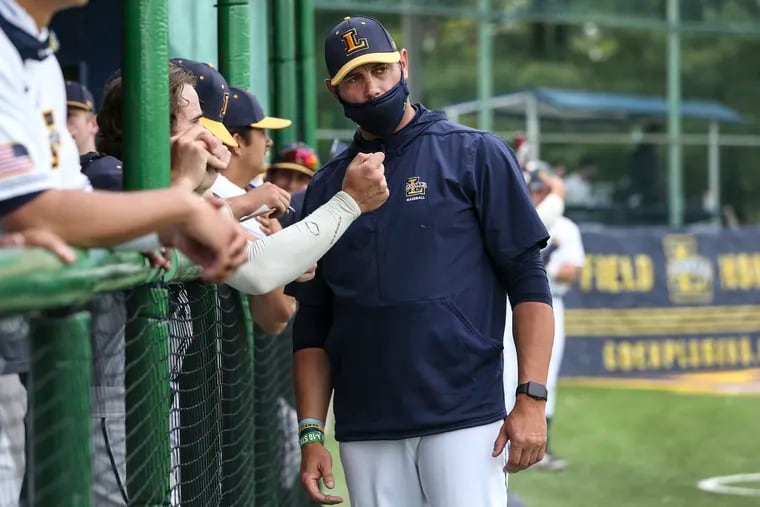The image captures an outdoor baseball scene, focused on a game field. On the left, there is a green fence, bordered by spectators. One spectator, wearing a long white-sleeved shirt, stretches his hand into the field area. Many observers, some of whom wear black baseball caps with yellow visors, stand beyond the fence. In the center, a man wearing a black baseball cap with an orange letter "L" on the front, stands prominently. He is dressed in a dark blue hoodie with a logo on its chest and white pants. This man also wears a black face mask. The background reveals a blurred banner with yellow text on a blue background and green trees. On the right side of the image, the edge of the playing field is marked by a white outline of one of the diamonds. The photo also hints at an American flag patch on one man's sleeve and a possible scoring stand with a blue roof. One individual, potentially the coach, is seen wearing a blue cap with an orange "L" and a yellow visor, a blue jacket, a black smartwatch, and colorful bracelets on his right wrist.